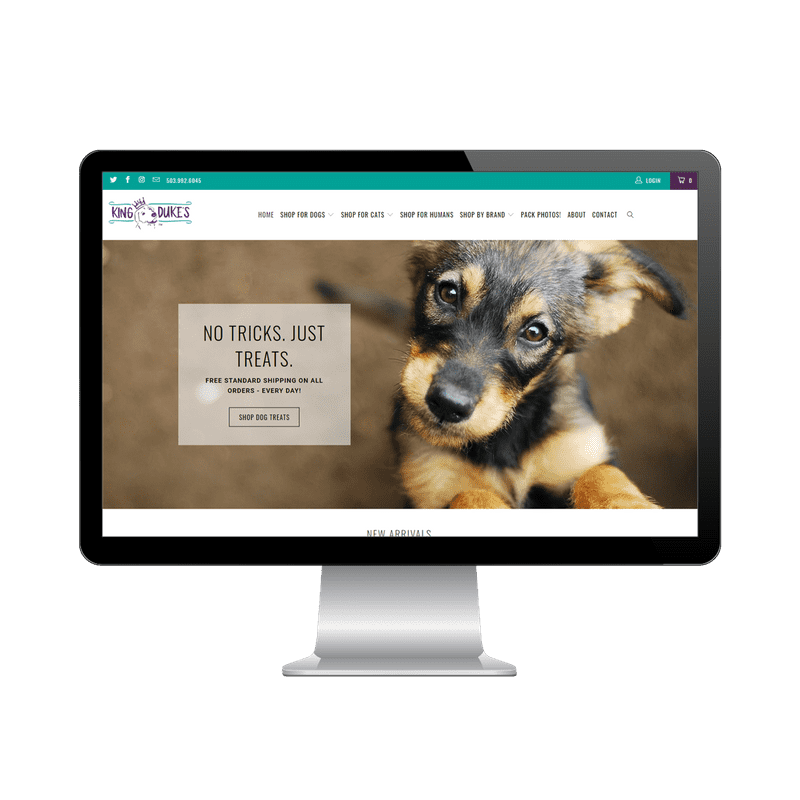The image depicts a website landing page primarily for pet-related products. At the top, there's a partially visible phone number next to a "Log In" option. Below that, there's a navigation bar with multiple tabs including "Home," "Shop for Dogs," "Shop for Cats," "Shop for Humans," "Shop by Category," "Photos," "Help Out," "Contact Us," and "Contact Dogs."

Central to the page is a prominent section featuring the text "King Dukes," accompanied by artwork and an image of a dog. There's also a conspicuous card that says "No Tricks, Just Treats" alongside a banner proclaiming "Free standard shipping on all orders, every day."

To the right, there's a highlighted call to action, "Shop for Treats," with an adjacent image of a dog adorably tilting its head. Additionally, there’s a section heralding a “New Arrival” with repeated prompts to "Watch this."

The page features an all-black border, contrasting sharply with a gray stand at the bottom which also has an emphasized line for delineation. The varied borders around different sections add an extra layer of distinctiveness to the page layout.